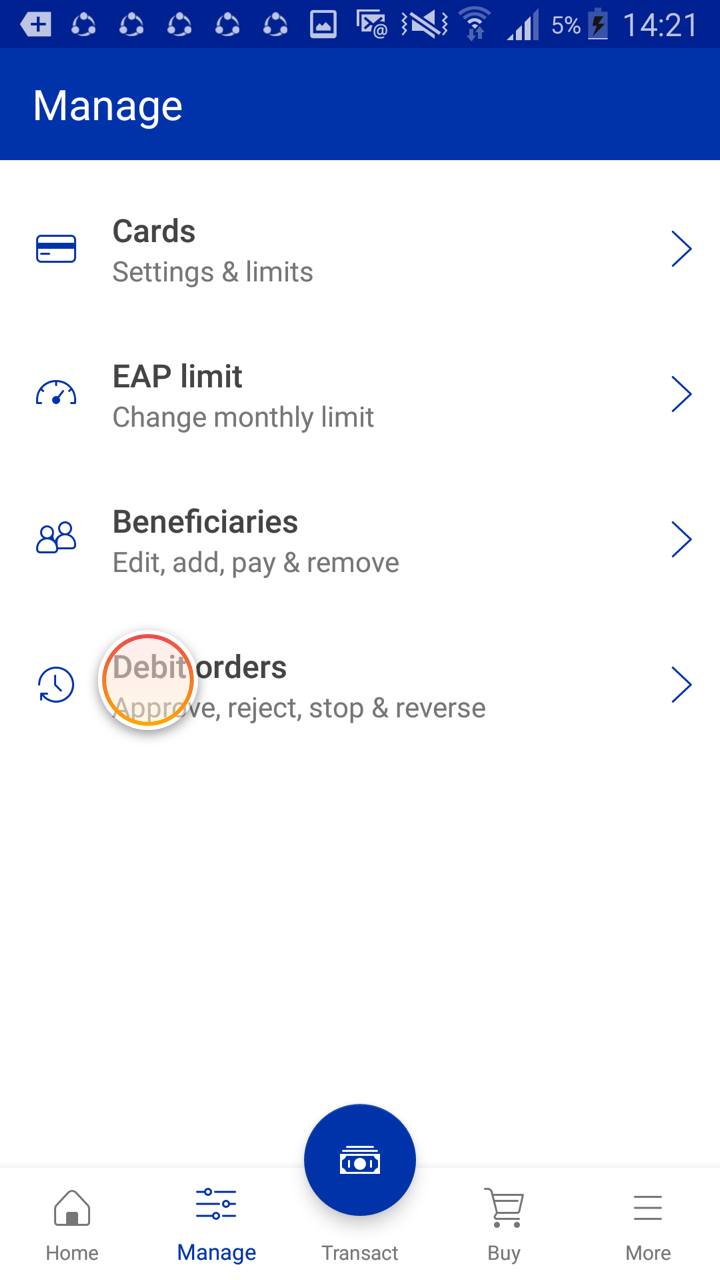The image depicts a screenshot of a cell phone display, showcasing a financial management app. At the top, there's a blue notification bar featuring a plus sign, a tag icon, and a series of five circular icons with dots inside. The bar also indicates an image icon, an email notification, and a symbol showing the phone is on vibrate mode. Additional details include information on connectivity, displaying Wi-Fi or data connection, cellular signal strength, a 5% battery level, and the time, which is 14:21. All these elements are depicted in white against the blue background.

On the left side of the blue bar, there is a "Manage" option. Below this, on a white background, are various sections with titles and corresponding right-facing arrows indicating further options. These sections include:

1. **Cards, Setting and Limits** - with a right arrow.
2. **EPA Limit, Change Monthly Limit** - with a right arrow.
3. **Beneficiaries, Edit and Add, Edit, Add, Pay and Remove** - with a right arrow.
4. **Debit Orders, Approve, Reject, Stop and Reverse** - with a right arrow.

A prominent feature includes a semi-transparent, red-orange circle with a peach tint over the "Debit Orders" section.

At the bottom of the screen are navigation options: **Home**, **Manage**, **Transact**, and **Buy More**. The "Transact" option is highlighted by a blue circle featuring a dollar sign or paper money symbol in white. The rest of the options are colored gray, with the "Manage" option also highlighted in blue. The right arrows in the upper sections are blue as well.